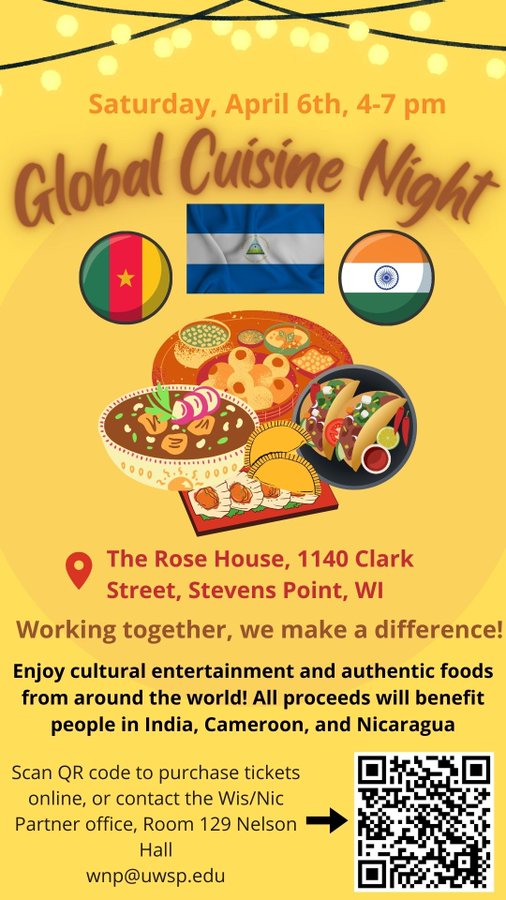The image is a bright yellow flyer advertising "Global Cuisine Night". At the very top, there is an illustrated string of lights. Just below, the flyer details the event date and time in yellow writing: "Saturday, April 6th, 4-7 PM". Centered below this, the title "Global Cuisine Night" is prominently displayed. Beneath the title are illustrations of three international flags, followed by clipart of various dishes including tacos, tabbouleh, sushi, and empanadas. 

The flyer also features a GPS pin icon with the event location: "The Rose House, 1140 Clark Street, Stevens Point, Wisconsin". Additional text reads, "Working together, we make a difference. Enjoy cultural entertainment and authentic foods from around the world. All proceeds will benefit people in India, Cameroon, and Nicaragua." At the bottom right corner, there is a QR code for purchasing tickets and getting directions, with further instructions to contact the WIS partner office at Room 129, Nelson Hall, WNP via the email uwsp.edu.

Bright and inviting, the flyer effectively communicates the details and purpose of the Global Cuisine Night event.